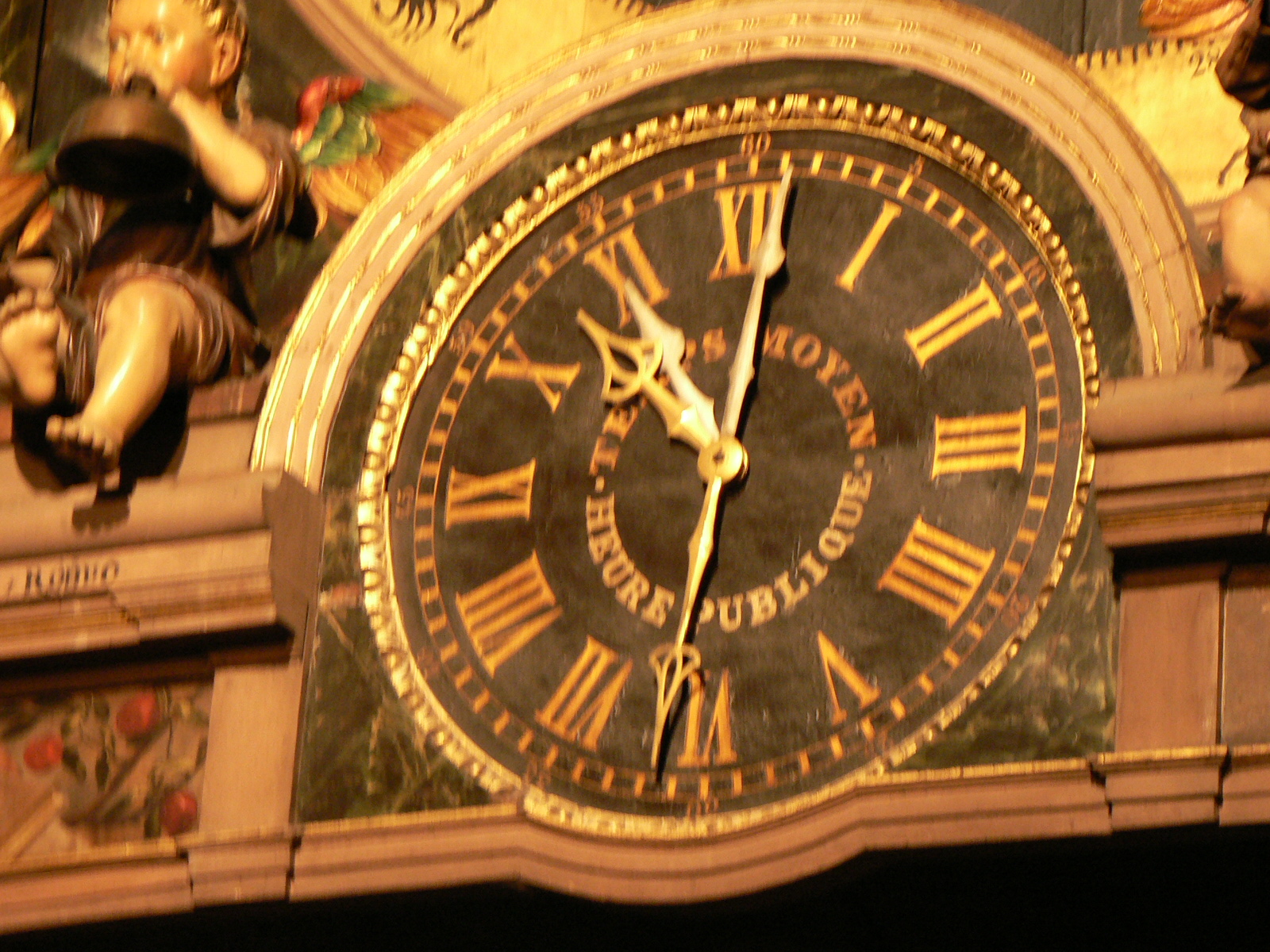The image features a decorative clock with a dark brown face and brass or gold arms positioned within an ornate architectural overhang, presumably part of a public transportation hub such as a bus or train station. The clock displays Roman numerals in yellowish-orange lettering and has four brass or gold hands showing two separate times. The clock is half-domed on top and framed by a gold band, with a circular, black background. The photograph has a warm, orangish filter, giving an overall yellow tint to the scene.

To the left of the clock, a detailed figurine of an angel with brown robes and rainbow-colored wings—red at the top transitioning to green and yellow feathers—is seen playing a rounded instrument or holding a wine flask. Below this, there are roses captured in a smaller framed picture. The shelf also holds a second figurine of a child gripping what appears to be a pot lid or cover. The intricate architectural details include elements of white arches and visible cement work around the clock.